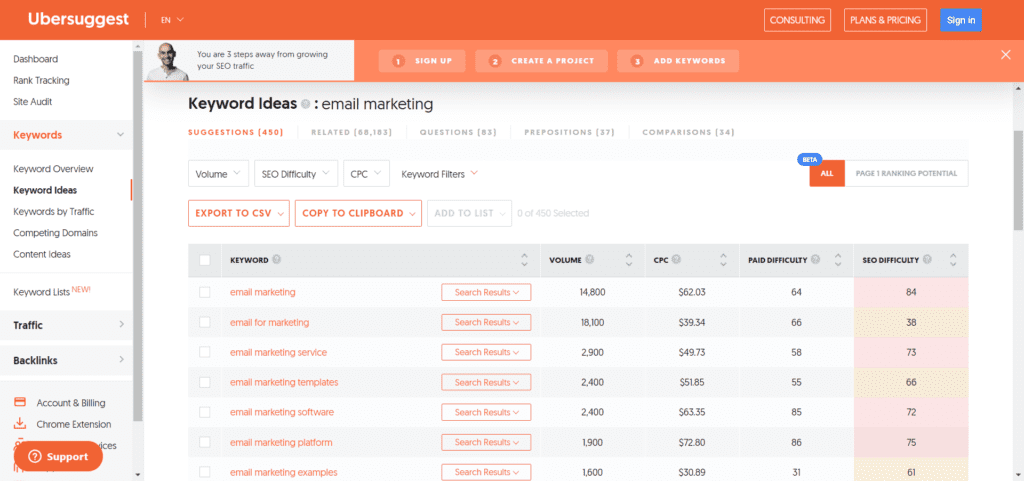This detailed screenshot depicts the interface of a webpage from UberSuggest, a digital marketing tool focused on enhancing SEO traffic. The layout initiates with a vertical menu on the left-hand side. An orange banner extends across the top of the page, prominently displaying the UberSuggest logo on the far left. Aligned to the right within this banner, three distinct buttons are labeled "Consulting," "Plans and Pricing," and "Sign In."

Beneath this banner resides a white box containing the image of a man along with a motivational message stating, "You are three steps away from growing your SEO traffic." Adjacent to this are three actionable buttons in slightly lighter orange: "Sign Up," "Create a Project," and "Add Keywords."

The central portion of the page focuses on providing "Keyword Ideas: Email Marketing," organized into five categories: Suggestions, Related Questions, Prepositions, and Comparisons. There is a feature for managing an email inbox, which offers options for exporting data to a CSV file or copying it to a clipboard. Notably, much of the font color within the email inbox section is orange. Additionally, there is a slider bar on the right-hand side for navigation within the page.